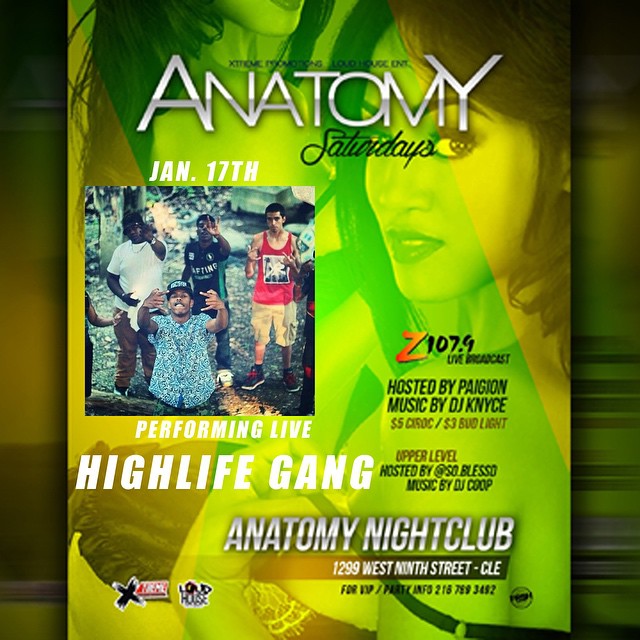The image is a vibrant and colorful promotional flyer for an event at Anatomy Nightclub. At the top, it prominently features the text "Extreme Promotions, Loud House Entertainment presents Anatomy Saturdays, January 17th." The main background displays images of women, one of whom appears to be wearing lingerie. To the left, there is a photograph of four men posing, each dressed uniquely—one in white, another in a blue shirt, the third in a green and black jersey, and the last in a red tank top. More text on the right side announces a live broadcast by Z107.9, hosted by Pagan, with music by DJ KNYCE. The flyer also advertises "Performing Live: High Life Gang" and offers a promotion of "$5 to rock, $3 Bud Light." The event is set to take place at Anatomy Nightclub, located at 1299 West 9th Street, CLE. The overall design is eye-catching with an array of colors including black, brown, tan, green, yellow, blue, and red.